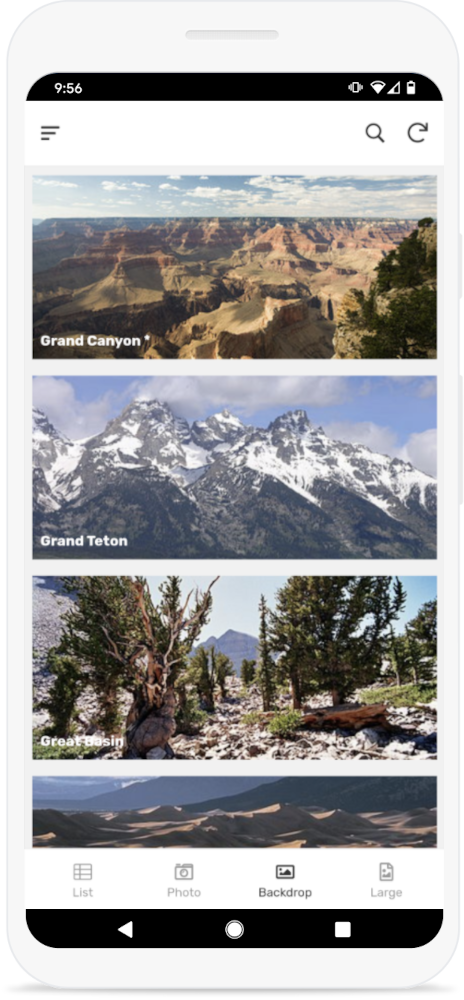The screenshot depicts a mobile interface with a white border that mimics the appearance of a phone screen. In the top left corner, it displays the time, "9:56," alongside mobile connectivity indicators, service bars, and a battery icon. Below the time, there are three horizontal lines representing a menu, followed by a search icon and a refresh icon.

The main body of the screenshot features a series of images. The first image captures the Grand Canyon, showcasing the intricate shapes of its inner walls with varying hues of brown and red, all set beneath a blue sky with scattered clouds. "Grand Canyon" is labeled in the bottom left corner of this image.

Below that, a close-up image of snow-capped mountains under a blue sky with clouds is labeled "Grand Teton."

Further down, an image displays trees with a distant mountain, labeled "Great Basin" in the bottom left corner.

Partially visible at the bottom is one more image that shows silhouettes of hills, though the location remains unspecified due to it being cut off.

Finally, at the very bottom of the interface, there are options labeled "List," "Photo," "Backdrop," and "Large."